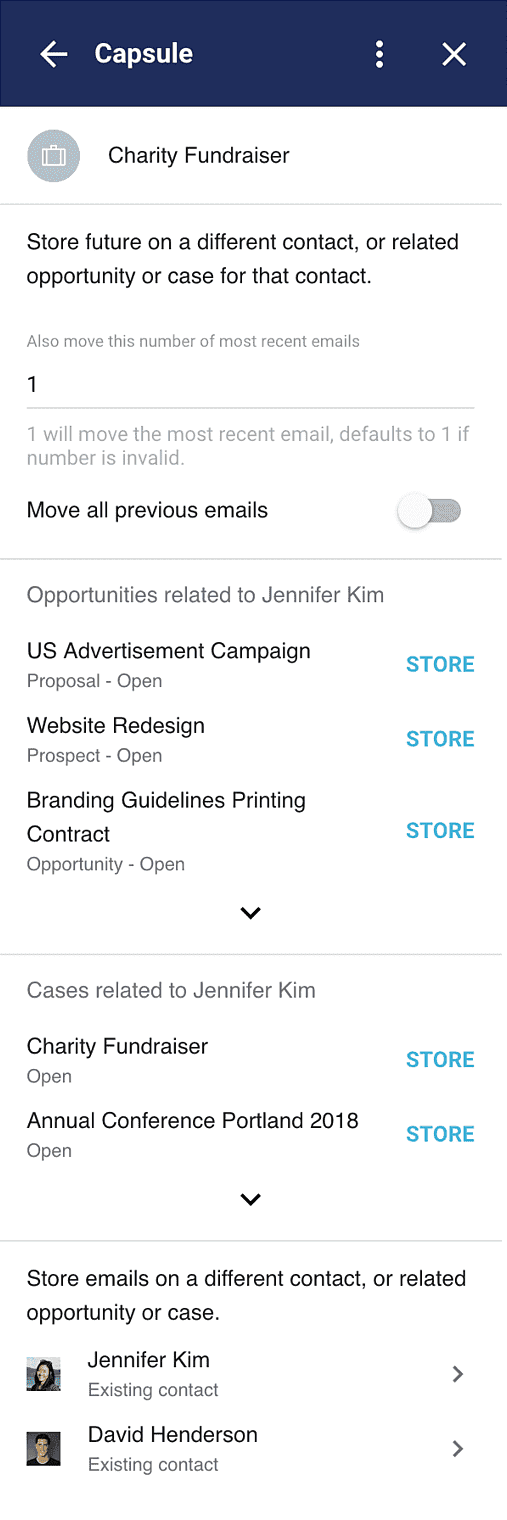The image depicts a webpage titled "Capsule" with a blue header bar. The word "Capsule" is prominently displayed in white font, accompanied by an arrow pointing to the left, three vertically aligned dots, and an 'X' icon. The top section is labeled "Charity Fundraiser," featuring a gray circle with a placeholder box image.

Beneath this, the content outlines several features and instructions. It mentions "Store a future on a different contact or related opportunity or case for that contact," followed by an option to "Remove the most recent email," which defaults to one if the number is invalid. There is a switch for "Move over previous emails," which is currently off.

The section "Opportunities related to Jennifer Kim" lists several entries:
- "US Advertisement Campaign" marked with a blue "Store" button.
- "Website Redesign," also with a blue "Store" button.
- "Branding Guidelines" and "Printing Contract," each accompanied by a blue "Store" button.

Following this, the section "Cases related to Jennifer Kim" lists:
- "Charity Fundraiser" with a blue "Store" button.
- "Conference Portland 2018" also marked with a blue "Store" button.

Lastly, the image shows profile pictures and names, indicating contacts. Jennifer Kim's profile is displayed as the existing contact on the left, while David Henderson's profile is shown on the right as another existing contact, connected by an arrow.